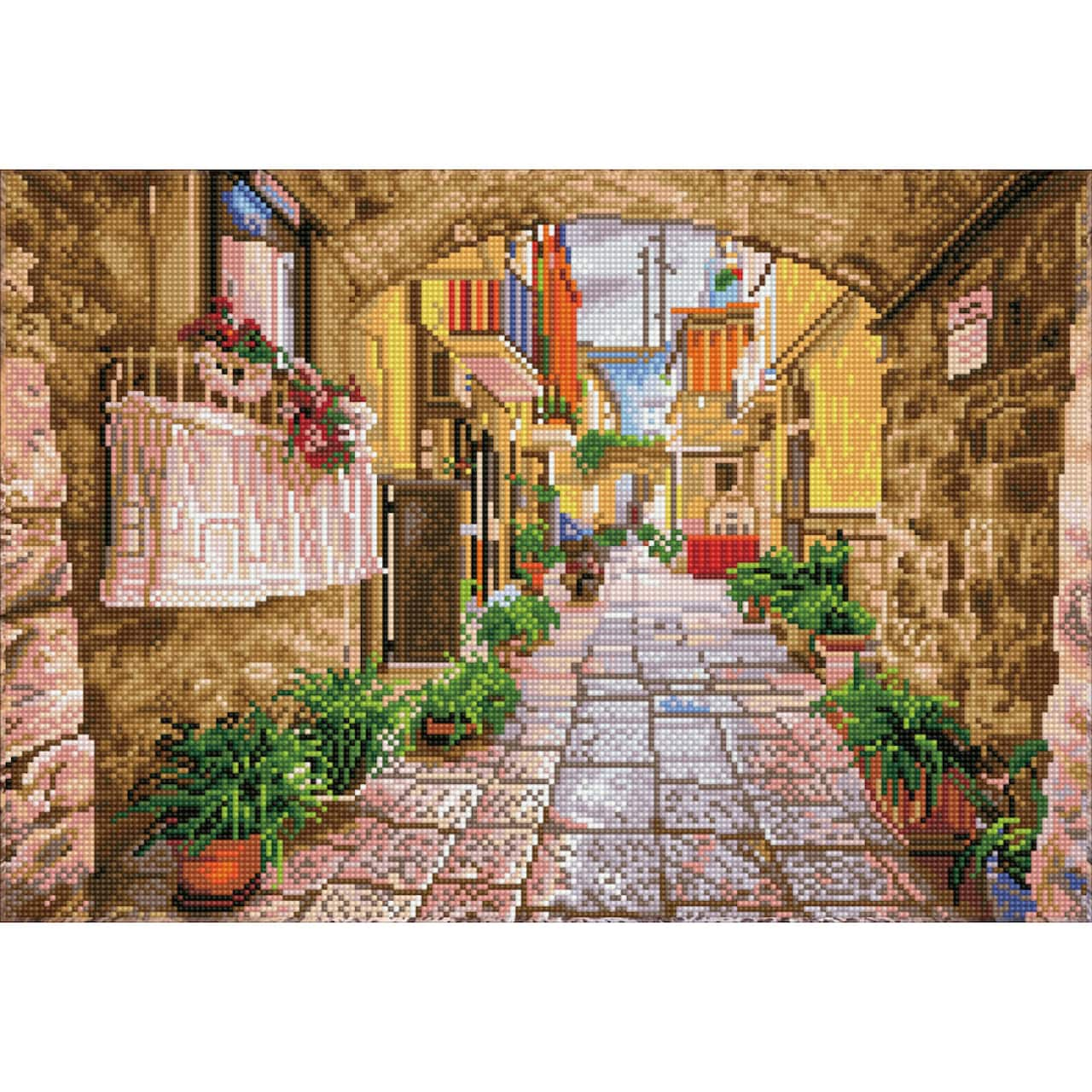This image showcases a vibrant pixel art scene reminiscent of early video games from the late 80s to early 90s. Set in a European-style cityscape, the focal point is a stone pathway composed of light purple, white, and light pink pixels that gradually narrows and disappears into the distance. Lined with several green potted plants in orange containers, the path leads between buildings adorned with balconies and archways. These buildings display a diverse palette of colors, including tans, golds, pinks, yellows, and oranges, creating a lively yet nostalgic atmosphere. Above, a soft, white-gray sky tinged with hints of purple adds to the overall charm, making the image appear almost like a meticulously crafted pixel puzzle.